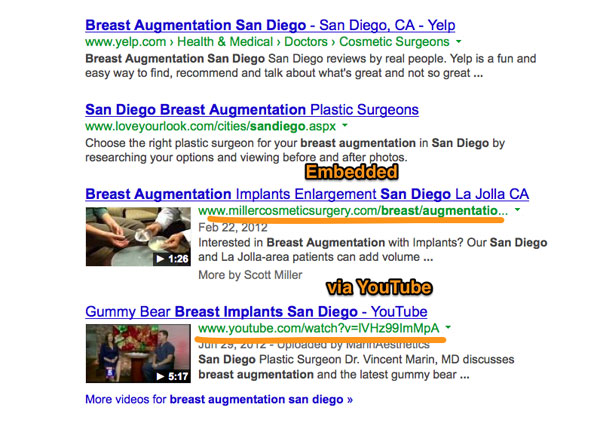The image depicts a Google search results page for the query "Breast Augmentation San Diego." The location specified in the search is San Diego, California. The first result is a Yelp page for "San Diego Breast Augmentation Plastic Surgeons." Further down, there's a listing titled "Breast Augmentation Implants Enlargement San Diego" in La Jolla, California, with the web address "millerscosmeticsurgery.com/breast/augmentation" highlighted in orange with the word "Embedded" above it. 

To the left of this listing, there's a video thumbnail labeled "Interested in Breast Augmentation with Implants" from YouTube, emphasized in orange text. Another search result below this one features a link to a YouTube video discussing "Gummy Bear Breast Implants San Diego," accompanied by a video thumbnail to the left. The page suggests additional videos related to "Breast Augmentation San Diego" at the bottom.
 
This well-structured caption provides clarity on the search result layout, highlights, and relevant information about breast augmentation options in San Diego, including multimedia resources.